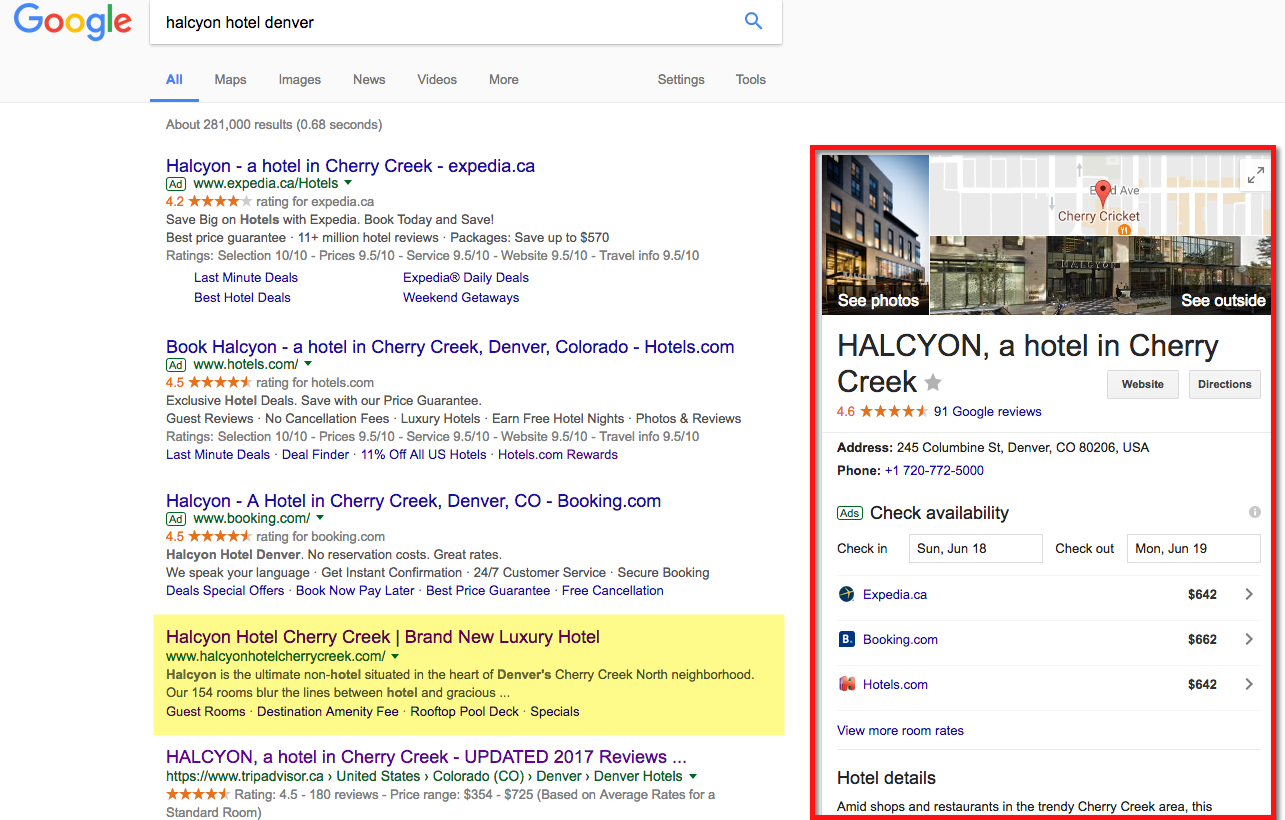The image depicts search engine results for "Halcyon Hotel in Cherry Creek, Denver." The top of the screen features a prominent information card about the Halcyon Hotel to the right, displaying detailed data like the hotel name, location (Cherry Creek), a 4.6-star rating based on 91 Google reviews, and a map. This card also includes the hotel's address, phone number, and an option to check availability, highlighting specific dates for check-in (Sunday, June 18th) and check-out (Monday, June 19th). Additionally, it shows various booking options with their respective prices: Expedia at $642, Booking.com at $662, Hotels.com at $642, and a link to view more rates.

On the left side of the screen, there are search results organized under various categories such as "All," "Maps," "Images," "News," "Videos," "More," "Settings," and "Tools." The "All" category is underlined in blue, indicating it is currently selected, while the other categories are in gray. The search results featured include links to booking sites like Expedia.ca, hotels.com, and cobooking.com, all listing information about booking the Halcyon Hotel in Cherry Creek, Denver, Colorado. Two additional unspecified search results appear at the bottom.